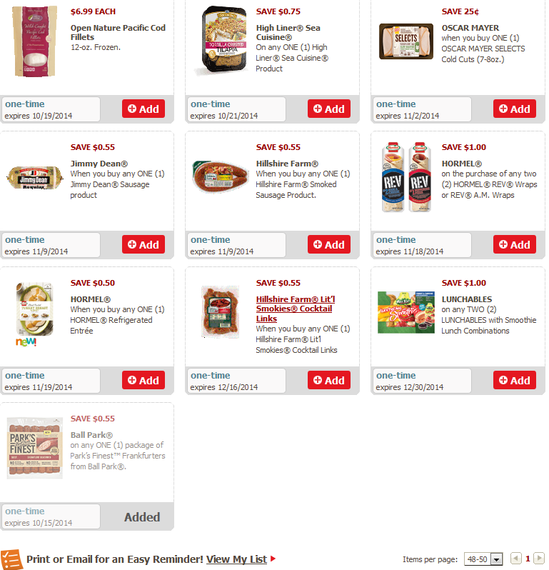The image displays a collection of discount items arranged in rows, available for adding to an online shopping cart. There are four rows in total, with the first three rows containing three items each, and the last row containing one item. 

1. **First Item**: Open Nature Pacific Cod Fillets, 12 ounces, frozen, priced at $6.99 each. The offer expires on October 19, 2020. There is a red "Add" button associated with this item.

2. **Second Item**: High Liner Sea Cuisine products, offering a discount of $0.75. The coupon can be used once and expires on October 21, 2014. This has a red "Add" button.

3. **Third Item**: Oscar Mayer Selects Cold Cuts, with a $0.25 discount. The coupon is valid for one-time use and expires on November 2, 2014. It also features a red "Add" button.

4. **Fourth Item**: Jimmy Dean Sausage products, available with a $0.55 discount. This offer is valid until November 9, 2014, and can be added to the cart with a red "Add" button.

5. **Fifth Item**: Hillshire Farm Smoked Sausage products, also discounted by $0.55. The one-time use offer expires on November 9, 2014, and has a red "Add" button next to it.

6. **Sixth Item**: Hormel Rev Wraps or Rev AM Wraps, with a $1 discount on any two purchased. This offer expires on November 18, 2014. Similar to the others, it includes a red "Add" button.

The detailed format allows shoppers to easily identify product details, prices, discounts, and expiration dates, all of which are clearly marked with actionable "Add" buttons for convenience.